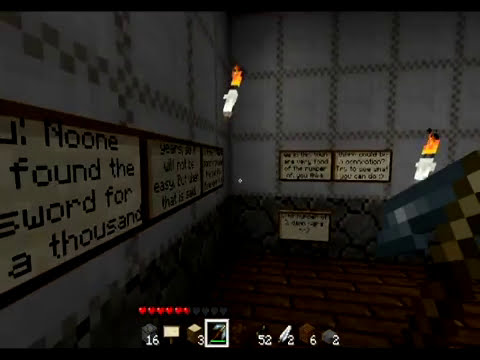In this pixelated, low-resolution video game scene, two small, Lego-like characters with yellow faces stand amidst a dimly lit environment, suggesting an 8-bit aesthetic reminiscent of Minecraft or Roblox. The setting features gray walls marked with a light brown grid pattern and blue sections outlined in black squares, lending a checkerboard appearance to some areas. On the far right of the scene, there's an object resembling stairs or an escalator, with one character halfway up a wall in the background, hinting at non-traditional game physics. 

Bright, flame-like lights in hues of white, yellow, and orange illuminate parts of the scene, with one particularly noticeable flame stationed beside a stairway. Text on the walls reads, "No one found the sword for a thousand years," suggesting a long-standing quest or challenge. Additional words, including "J. Moon found the sword for a thousand," appear towards the far left but fade into the corner, becoming unreadable from the given perspective.

The floor is composed of brown bricks, complementing the lower parts of the gray stone walls. At the bottom of the screen, typical game interface elements display the player's stats: six hearts, indicating life or strength, with five filled and one half-filled, alongside several numeric icons that likely represent various resources or accomplishments, including the numbers 16, 3, 52, 2, 6, and 2 in different rectangular and cubular boxes. The overall color palette is dominated by shades of brown, white, yellow, red, gray, and blue, creating a cohesive yet complex visual impression.